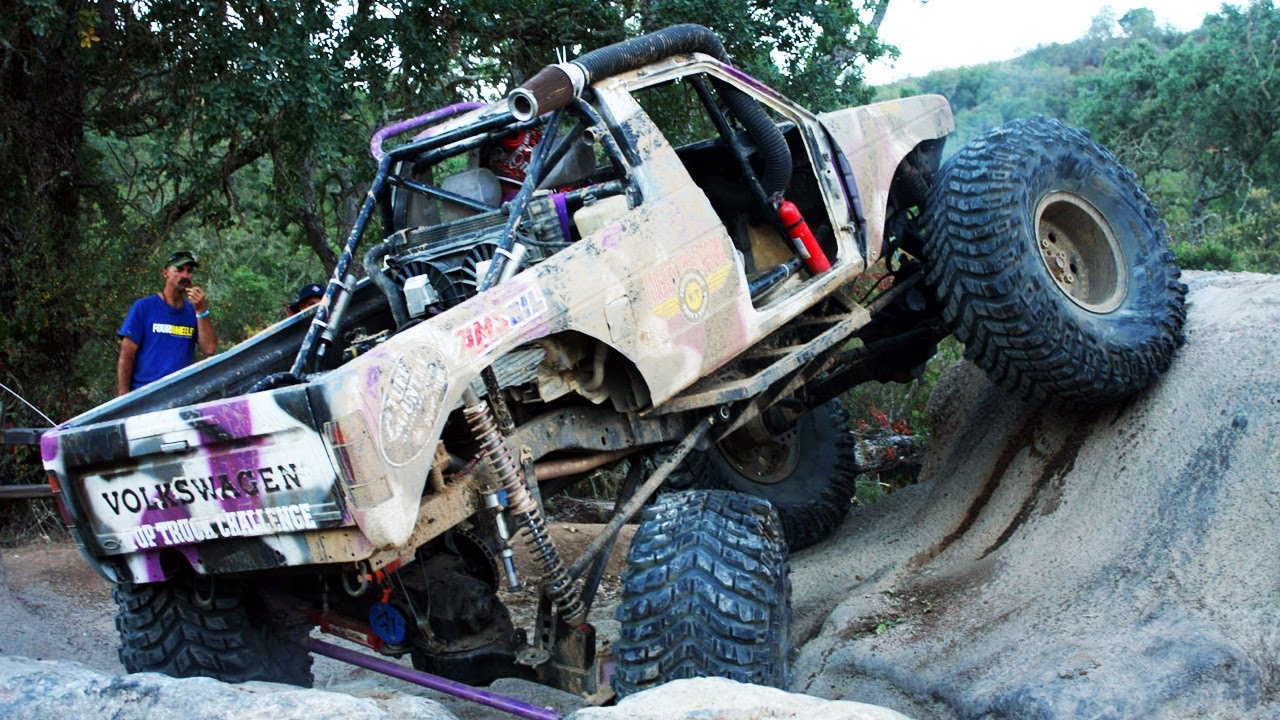The photograph showcases a Volkswagen monster truck engaged in an off-road challenge, evidenced by the "Up Truck Challenge" text prominently displayed on its tailgate. The truck, covered in dirt and mud, sports a tan color with enormous black tires that lift it high enough to expose its underside, including the suspension rods. Positioned halfway up a rugged rock formation, the vehicle appears to be stuck, with its back right tire bent and seemingly broken. A man in a blue t-shirt and green hat stands beside the truck, his hand to his mouth in a gesture of concern. The background features a dense array of green trees under a clear white sky, adding to the rugged outdoor setting of the scene.